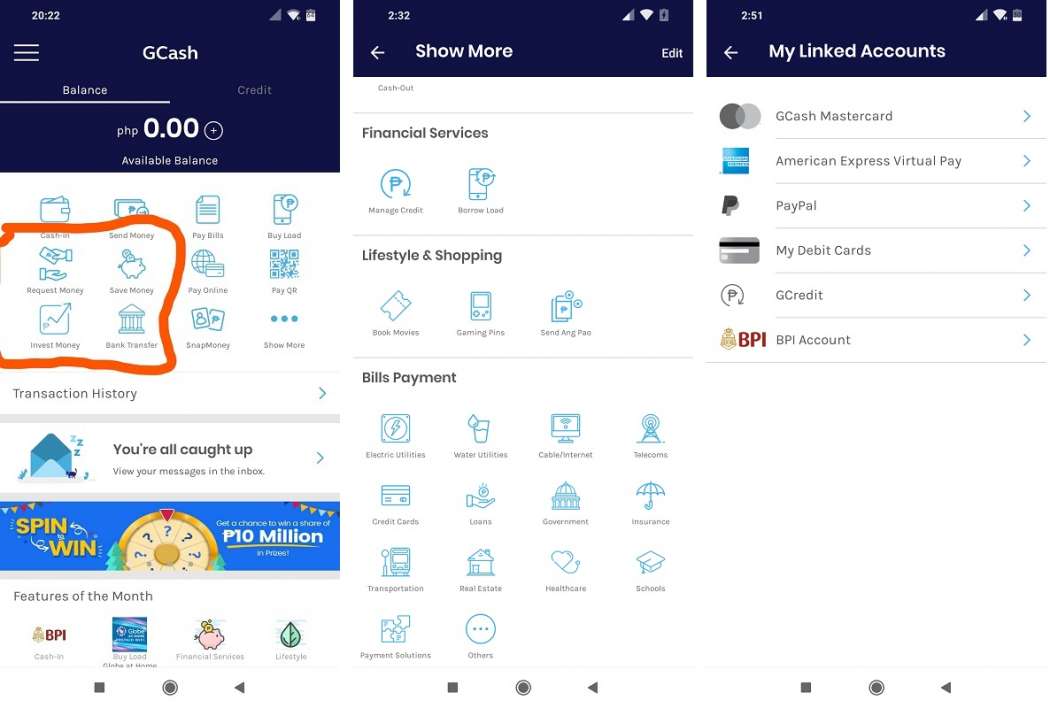This image showcases three cell phone screens arranged from left to right, each displaying different sections of a mobile app interface.

On the left screen, the top left corner shows the time as 20:22, accompanied by a connection icon, Wi-Fi icon, and battery life icon on the right. Below this status bar is the app's title, "GCache," with a menu icon consisting of three lines to its left. Underneath, the interface displays "Balance" on the left with "Credit" on the right, and "Balance" is selected, indicated by an underline. Below the balance number, there are 12 blue categories, with the four bottom-left categories highlighted in orange. Following this section is the "Transaction History" label, below which it says "You're all caught up." At the base of this screen, there is a game advertisement, and four icons are positioned at the bottom.

The middle screen shows the time as 2:32 in the top left corner with the same connection, Wi-Fi, and battery icons on the right. Below, the interface has a "Show More" option, followed by sections labeled "Financial Services," which has two options, "Lifestyle" with three options, and "Shopping" with three options. Additionally, there is a "Bills Payment" category listing 14 options in light blue.

The right screen displays the time as 2:51 in the top left corner, with the usual icons on the right. The main content starts with "My Linked Accounts" in white, followed by six categories. The common aesthetic feature across all three screens includes a dark blue, nearly black background at the top, with the remaining parts of the screens in white.

At the bottom of each screen, there are three navigation icons: a square on the left, a circle in the middle, and a sideways triangle pointing to the right.